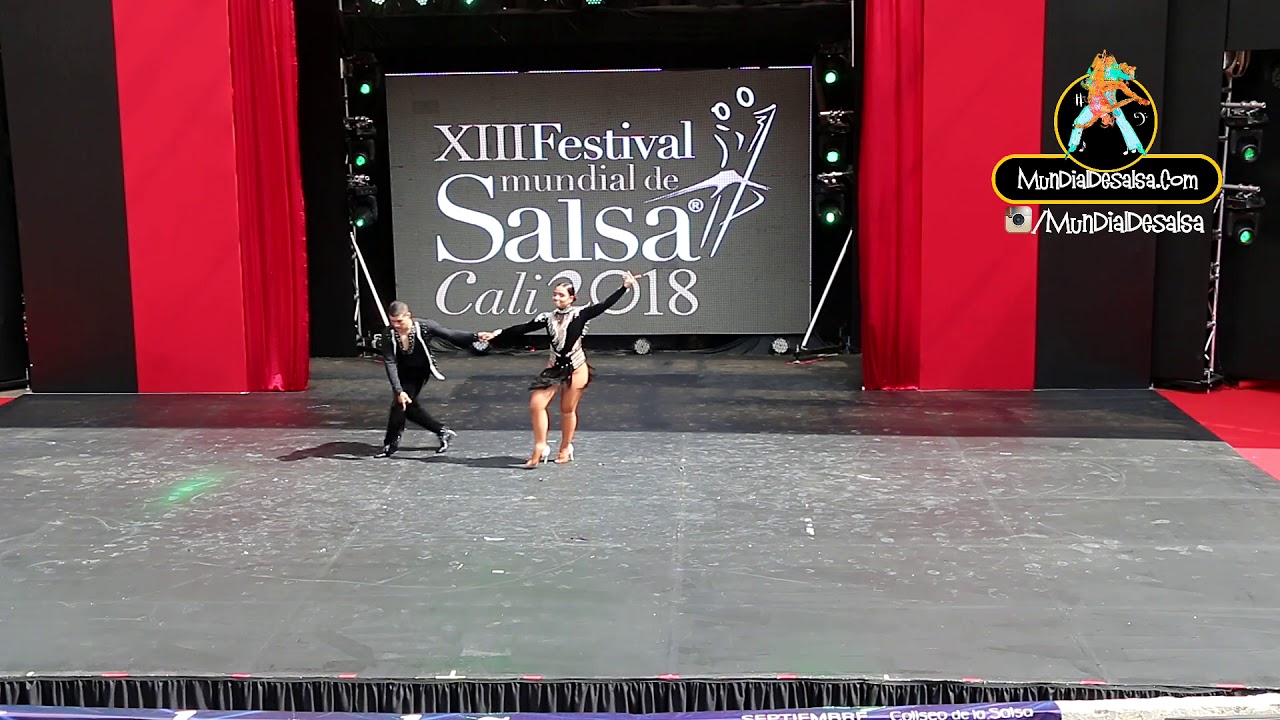The image captures a vibrant moment from the 13th Annual Festival Mundial de Salsa, held in Cali in 2018. At the heart of the scene are two dancers on stage, performing a salsa routine with elegance and grace. The man, dressed in a sleek black outfit, is bowing forward while holding hands with the woman to his right. She wears a short black dress complemented by striking pink high heels. 

Behind them, a large sign boldly announces the event with the text "XIII Festival Mundial de Salsa" in white font against a dark gray backdrop. The stage setting is dramatic, with towering red curtains framing the sign on both sides, while black curtains add depth to the outer edges. Noticeable in the top right corner of the scene is a logo depicting a dancer in turquoise pants, bordered in a yellow frame that also includes the website "mundialdesalsa.com" and its Instagram handle. Additionally, green stage lights cast a glow near a pole on the right side, where the floor transitions to a red hue, enhancing the lively atmosphere of the festival.